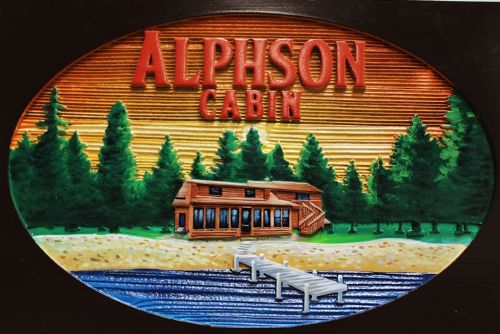The image titled "Elphicine Cabin" is depicted on an oval-shaped, raised wooden plaque or sign. In bold, red lettering at the top, the words "Elphicine Cabin" are engraved, standing out prominently against the intricate line patterns of the background. The background transitions from a brown hue at the top to yellow below, with a landscape featuring tall, green, triangular pine trees surrounding a brown cabin. The cabin itself is detailed with three windows on the second floor and eight rectangular windows on the ground floor, centered around a main entrance. An additional staircase to the right ascends to the second floor. In the foreground, a blue river extends across the scene, with a small white platform or pier reaching out from the shore, connected by a pathway leading directly to the cabin's front door. The scene is enriched by a green grassy area beneath the trees, contrasting with a yellow shore that meets the blue water below, completing the picturesque setting of the "Elphicine Cabin".